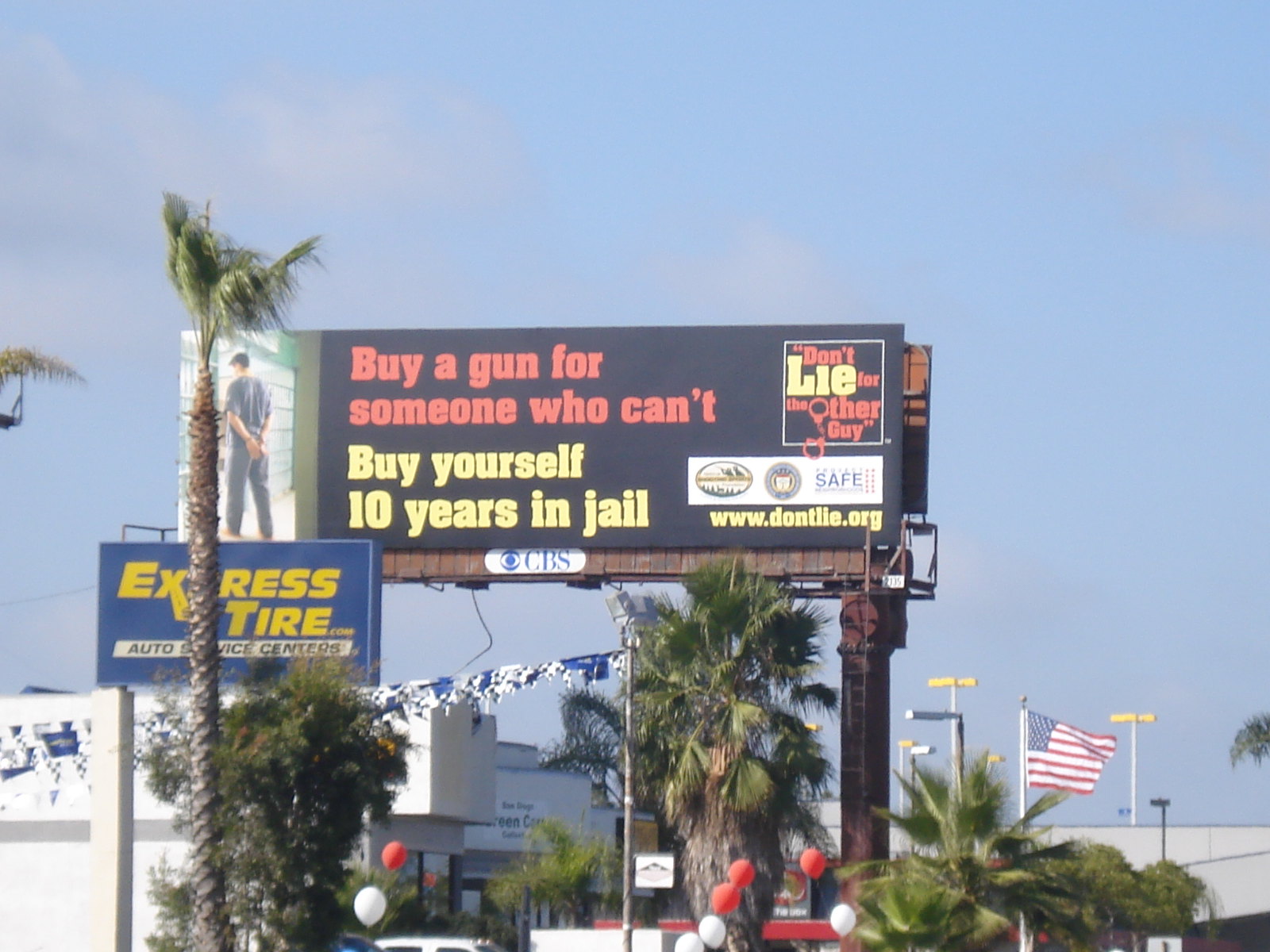The photograph captures a billboard located along a highway, likely taken in a tropical setting such as Florida or California, as evidenced by the cluster of tall palm trees in the vicinity. The image features a sunny daytime backdrop, characterized by a blue sky with scattered wispy clouds and an American flag fluttering off to the right. Below the billboard, red and white helium balloons can be seen, along with the tops of automobiles, suggesting the presence of a nearby auto mall or car dealership.

The primary billboard displays a stark message in bold red letters: "Buy a gun for someone who can't." Directly beneath this, in contrasting yellow text, it warns, "Buy yourself 10 years in jail." A visual of a person in handcuffs is positioned to the left of the billboard. To the right, there is a white box containing the phrase "Don't lie for the other guy," with "lie" highlighted in yellow and the remaining words in red. Below this phrase, a white rectangular box showcases various logos, and the web address "www.dontlie.org" is prominently displayed in yellow text.

In front of this prominent billboard, another sign reads, "Express Tire Auto Service Centers," with a palm tree partially obscuring it. Additionally, a blue CBS logo with a circular white detail is visible in the background, along with white and blue flags hanging between two silver poles.